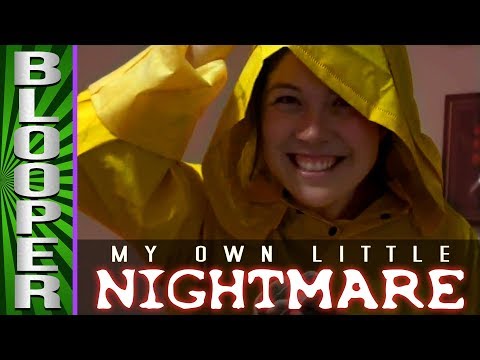The image is an indoor, digitally altered piece featuring a woman in a bright yellow raincoat with the hood up, smiling and raising her right arm. In the background, there's a black border that outlines the photo. On the left side, a light and dark green striped swirl runs vertically, with the word "Blooper" in white letters. Centrally positioned, the woman's picture is framed by black borders, with the phrase "my own little" in white text above a light red, neon-style "nightmare" written horizontally across her chest area. The woman, who has brunette hair and a white complexion, embodies the focal point of this visually striking composition that juxtaposes cheerful imagery with the caption "My Own Little Nightmare."